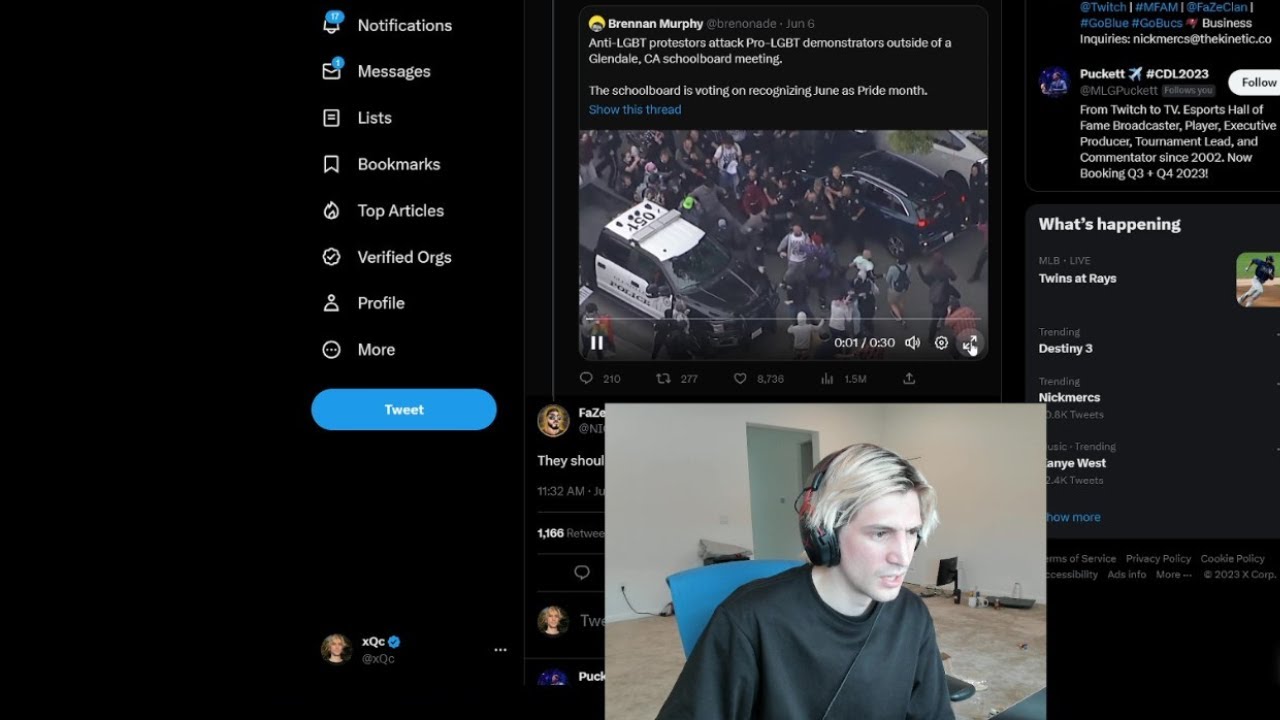The image features a black background with various elements. On the right side, there is text describing a video by Brennan Murphy, highlighting an incident where anti-LGBT protesters attacked pro-LGBT demonstrators outside a Glendale, California, school board meeting. The meeting's agenda includes voting on recognizing June as Pride Month. Below this description, there is a blue hyperlink labeled "Show this thread."

Further down, there's a section for business inquiries, referencing Puckett, with the identifier CDL 2023. It showcases credentials such as Twitch.tv eSports Hall of Fame broadcaster, player, executive producer, tournament lead, and commentator since 2002. It mentions availability for bookings in Q3 and Q4 of 2023.

Accompanying this text is an image of an individual with blonde hair, wearing headphones and a long-sleeve black shirt, seated in a blue chair. The room appears unfurnished with brown carpet, white walls, a gray door, visible cables emerging from the wall, and a computer monitor.

On the left side of the image, there is a sidebar containing various sections labeled Notifications, Messages, Lists, Bookmarks, Top Articles, Verified, Profile, and More. A blue button at the bottom is labeled "Tweet."

To the right, another sidebar titled "What's Happening" includes "Destiny 3" as a current topic.

This detailed caption encapsulates the essence of the image, noting both the visual and textual elements present.